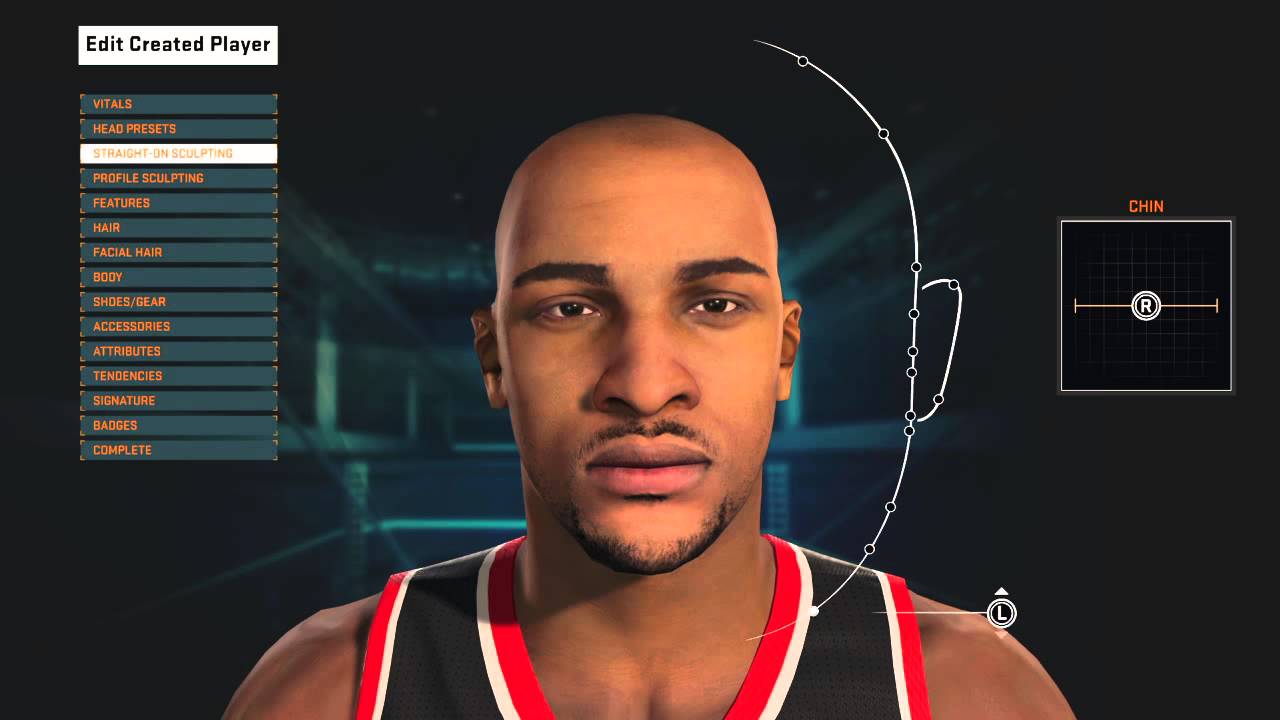The image, set in landscape orientation, appears to be a screenshot from a laptop. The background is predominantly dark green, shifting to a lighter green at the center, giving the impression of a light source. The image is a digital drawing featuring various interface elements. 

In the upper left-hand corner, within a white rectangle, the text reads "Edit Created Player." Below this header, a vertical list comprising 15 rows is visible. These rows are labeled as follows: Vitals, Head Presets, Straight On Sculpting (highlighted in white), Profile Sculpting, Features, Hair, Facial Hair, Body, Shoes, Gear, Accessories, Attributes, Tendencies, Signature, Badges, and Complete. While the highlighted "Straight On Sculpting" is in gold font, the other labels are in a dark orange font. The background of the menu items retains the dark green palette, accented with small hints of orange.

In the center of the image, a character being edited is displayed. The character is a dark-skinned man surrounded by a white outline dotted with small black dots, indicating editable points. He is attired in a black basketball team t-shirt featuring white stripes and a red collar. The man is bald and sports a mustache and goatee.

On the right-hand side of the image, a square interface element displays the label "Chin" in red. Various adjustment circles are present within this interface element, including one at the center and another at the bottom. Additionally, just above the character’s left shoulder, there is an "L" within a circle, signifying another editable feature.